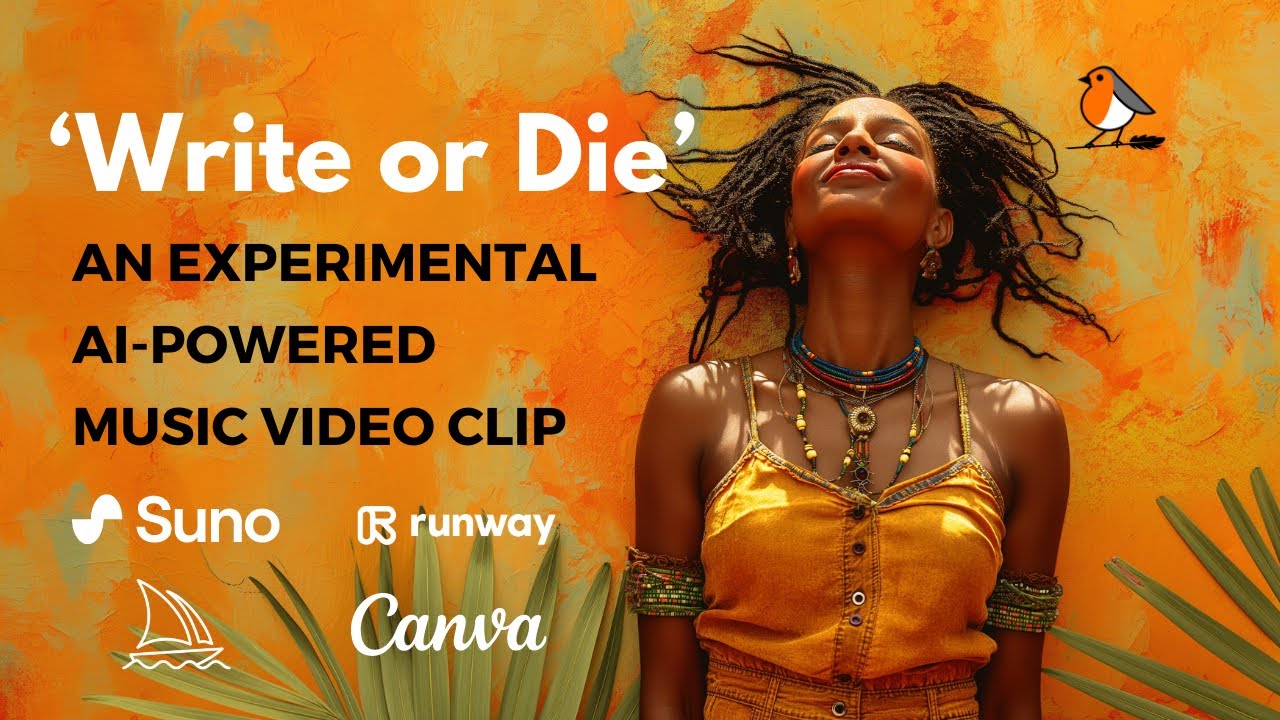The poster features a captivating blend of vibrant photography, illustration, and text. The background is a vivid mottled orange wall with intriguing olive green splotches. Positioned at the bottom center and right are pale green, fern-like leaves, delicately fanning out. Nestled between these plants is an African American woman, her face uplifted in a serene, sunlit smile. She dons an orange denim tank top tucked into matching denim pants, accented with dark green trim. Her forearms are adorned with green bands, detailed with white, red, and blue beads, and her neck showcases an array of intricate necklaces featuring blue, red, and white beads. Metallic earrings add a subtle shine, and her thin dreadlocks fan out gracefully across the surface. To the right of her, a cartoon-style bird with a red front, white belly, and black legs adds a whimsical touch. On the left side of the poster, in bold white text, it reads "Write or Die," followed by "an experimental AI-powered music video clip" in black. Below this, several logos are displayed: Suno, Runway, Canva, and a sailing boat illustration in white.